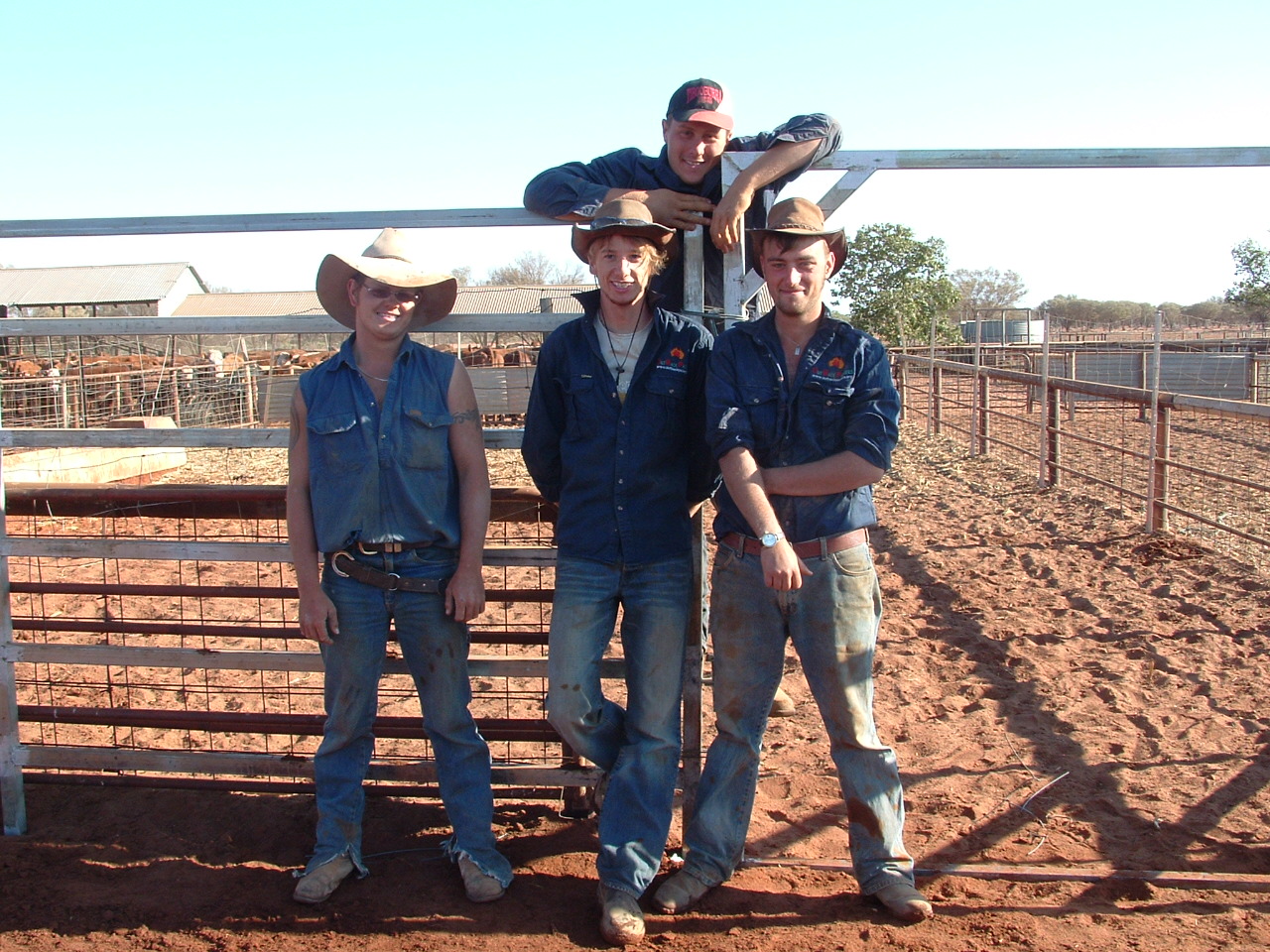The photo, taken outdoors on a bright, sunny day with a clear sky, features four younger males who appear to be farmers or ranchers. They all wear traditional cowboy outfits consisting of jean shirts and jeans, with three donning cowboy hats and one in a regular cap. The soil in the area is a distinct red, suggesting it might be iron-rich. These men, likely related due to their similar appearances, stand in front of a ranch enclosure. In the background, dozens of cows can be seen, along with a sandy ground, several short trees, and a water storage tank, contributing to the clear impression that this scene takes place on a farm.